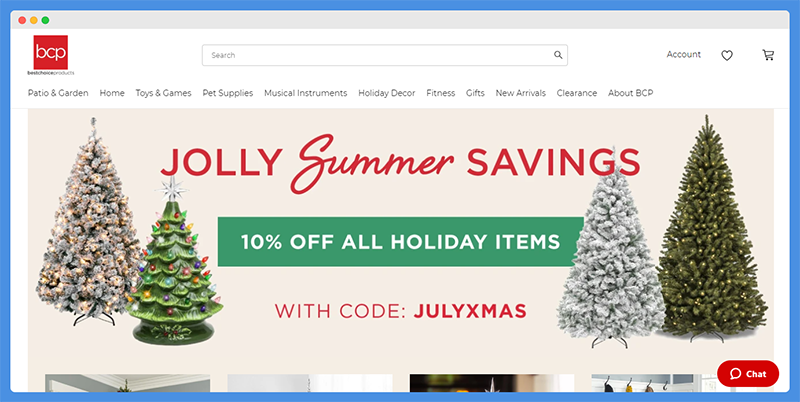This image captures a holiday-themed e-commerce website designed with a festive and visually appealing layout. The entire website is framed with a medium blue border, which sets a calm and inviting tone. At the top of the site, there's a beige banner featuring three colored circles—red, yellow, and green—positioned on the left side, possibly representing website controls or status indicators.

Beneath the beige banner, a white banner is displayed prominently. It contains a red square with the text "BCP" at the top left, alongside a centrally located search bar. On the far right of this banner, icons labeled "Account," "Favorites" (represented by a heart), and "Shopping Cart" are readily accessible for user interaction.

The main navigation bar below this banner lists various categories in an easy-to-read format: Patio and Garden, Home, Toys and Games, Pet Toys, Musical Instruments, Holiday Decor, Fitness, Gifts, New Arrivals, Clearance, and About BCP.

Further down the page, festive graphics emphasizing holiday cheer are showcased, featuring different kinds of Christmas trees—a ceramic one, a large snow-tinted tree, a fully decorated Christmas tree, and a green tree adorned with lights. Accompanying these visuals is a green banner proclaiming "10% off all holiday items."

At the very top of this section, a larger banner announces "Jolly Summer Savings," with a promotional message below that says you can get discounts using the code "JulyXmas," creating a sense of urgency and excitement for holiday shopping, even in the off-season.